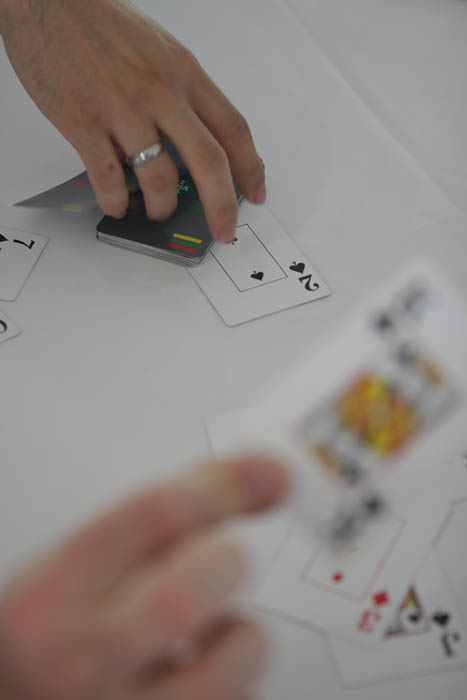This photograph captures a moment of an intense card game. The image is oriented in portrait mode and exhibits a blur towards the bottom section, adding a sense of dynamic ambiance. In the upper left-hand corner, we see a light-skinned person using their right hand to grasp an object—it's black and positioned atop a white card, possibly the deck's backside, featuring a design of black with yellow, green, and red stripes. The person's hand is adorned with a silver band ring on their third finger (commonly referred to as the fourth finger). This individual appears to be holding a two of spades card, while the seven of spades peeks slightly from the left side.

In the bottom left-hand corner, another light-skinned hand is in motion, seemingly placing a high-ranking card, likely a king, onto the table. Meanwhile, the bottom right-hand corner of the photograph clearly displays a jack of spades and a three of diamonds lying on the table. The game being played remains unidentified, but the players' intense concentration is palpable through every pixel of the image.